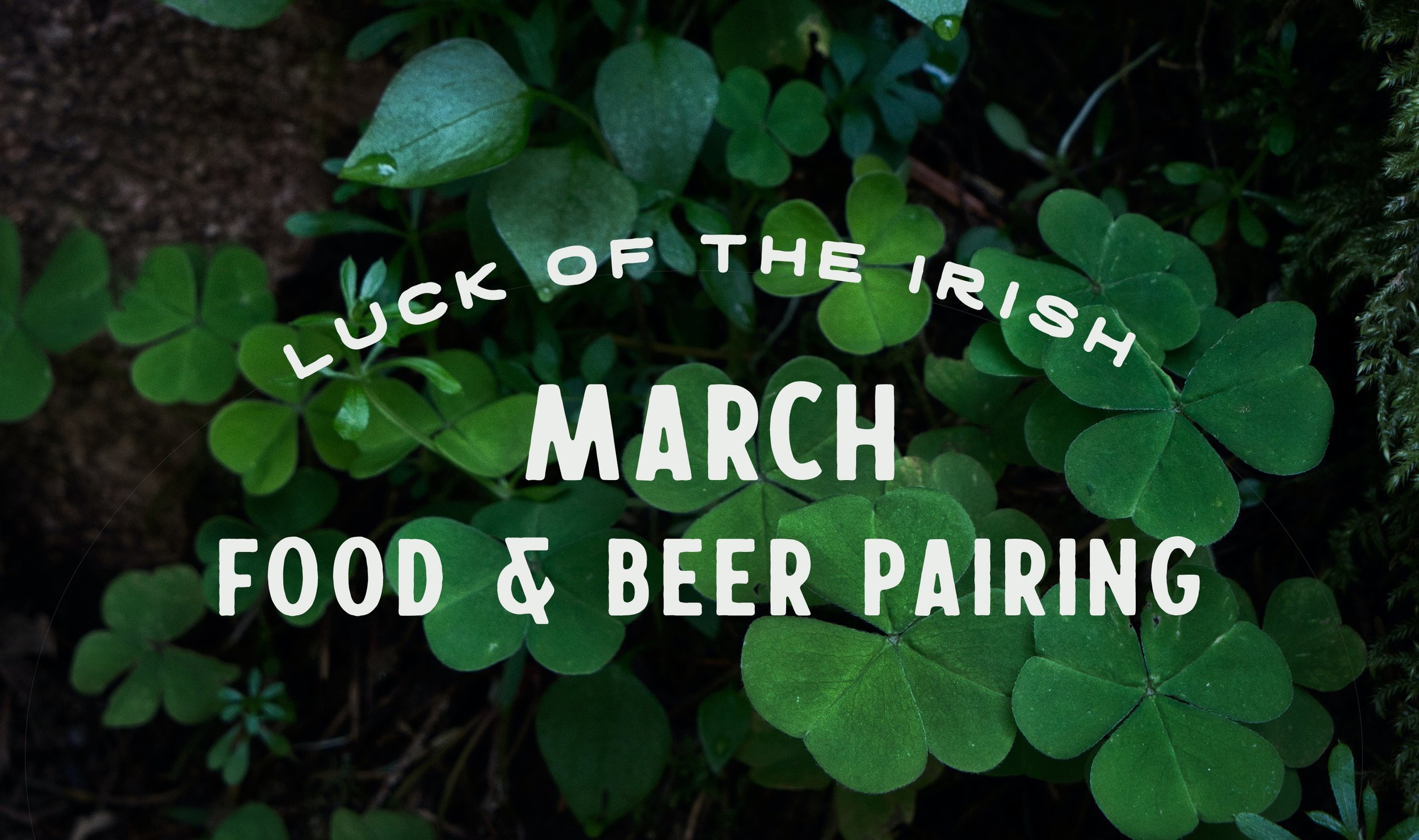This is a horizontal digital or printed promotional image with a dark background showcasing an overhead view of lush greenery. Scattered throughout are over 20 green shamrocks and clovers, including a mix of three-leaf and four-leaf varieties, and other green-leafed plants sprinkled with droplets of water. The vivid green hues of the plants against the dark background highlight a St. Patrick's Day Irish theme. At the center of the image, an arched white sans-serif font reads "Luck of the Irish," and below it in a similar white font, "March Food and Beer Pairing" is displayed, likely advertising an upcoming event at a restaurant or bar.